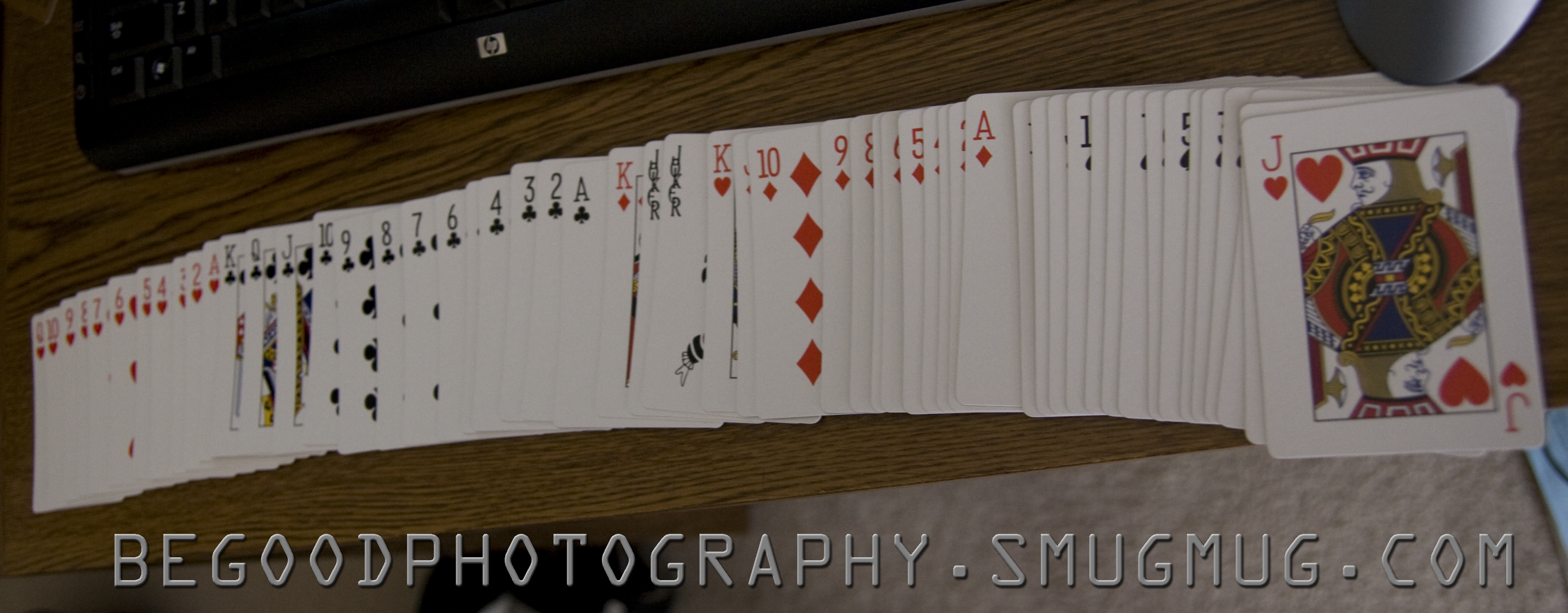On a richly textured, brown wooden desk with dark brown patterns and green lines, a close-up image captures a meticulously arranged deck of playing cards. Near the top left, the edge of an HP laptop with its keyboard area is visible, hinting at an ongoing electronic activity. Lined up neatly like dominoes, the entire deck of cards is displayed face-up, each card leaning against its neighbor. The arrangement culminates on the far right with a prominently featured Joker of Hearts at the top, adding a playful yet orderly touch to the scene.